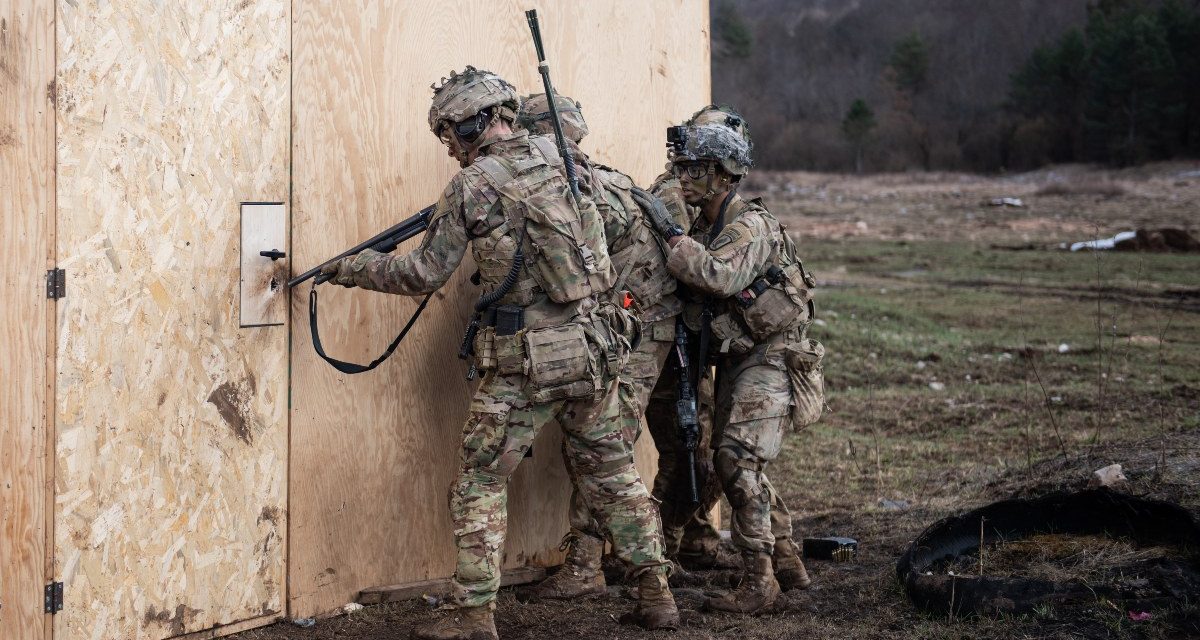In this image, several soldiers in full battle gear are depicted in what appears to be a training exercise, standing outside a temporary plywood structure. The building, constructed of light-colored plywood, and the door, made of OSB with metal hinges and a small metal handle, set an improvised scene typical of training simulations. Three soldiers are immediately visible: the one at the forefront is aiming his rifle at the door handle, seemingly having shot it to breach the door. Behind him, a second soldier is partially obscured but visible, with one hand resting on the back of the soldier in front. The third soldier, positioned just behind these two, has his hand on the second soldier's back and is watching intently. The scene is set outdoors, under an overcast sky, suggesting a gray, perhaps dreary, day. The ground is littered with debris, including old tires, adding to the realism of the training environment.